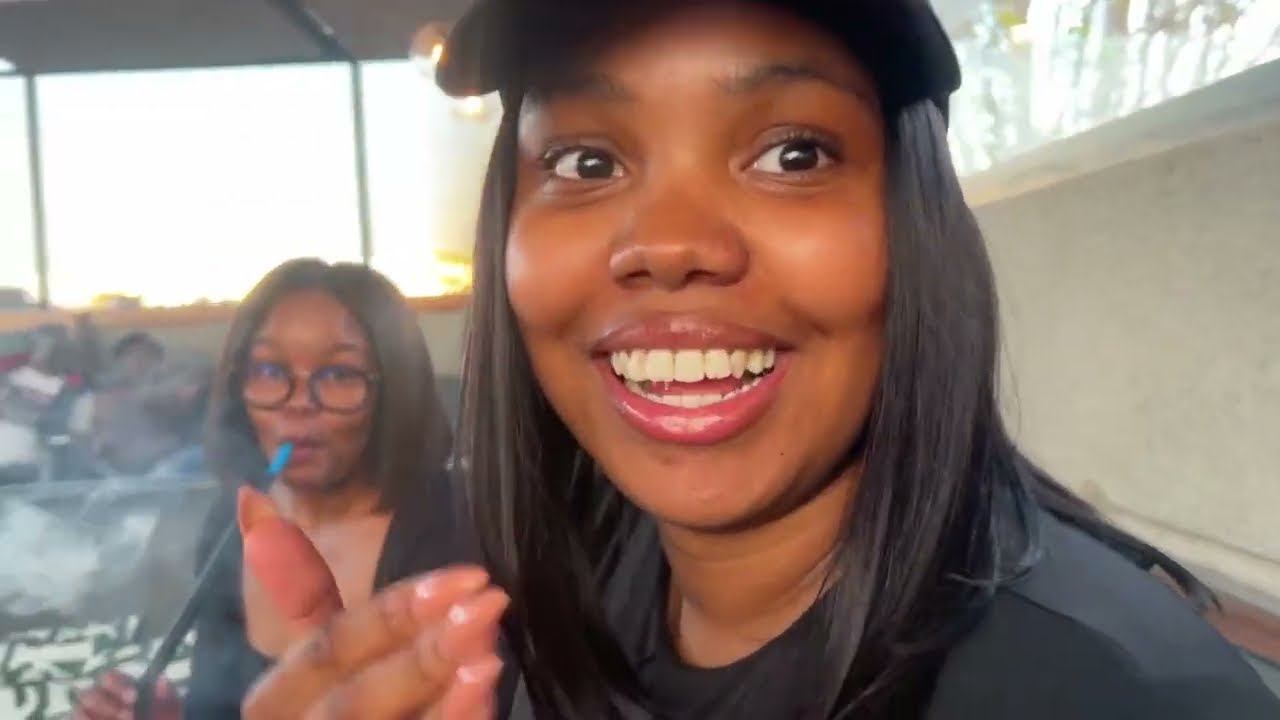In this rectangular, horizontally-oriented photo, two Black women are featured in an outdoor setting, likely a patio with a half wall enclosure and a large open window in the background allowing light to flood through, glowing softly. The primary subject is a smiling woman with big brown eyes, wearing a black baseball cap atop her straight shoulder-length black hair. She’s dressed in a black shirt and gesticulating with her right hand, which is adorned with sharp, pink-painted fingernails. Her mouth is open, revealing her top row of teeth and her tongue beneath them, giving the impression that she is speaking or laughing.

Behind her, to the left, stands another Black woman with shoulder-length hair, wearing circular-rimmed eyeglasses. She holds a black stick, possibly a hookah tube, which changes to a light blue color where it enters her mouth, enveloped by a slight smokiness. The scene captures a lively and joyful moment shared between the two women, with the bright, glowing lighting from the background window accentuating their expressions and creating a warm, engaging atmosphere. The white wall on the right side frames the setting neatly, contributing to the overall composition of the photograph.